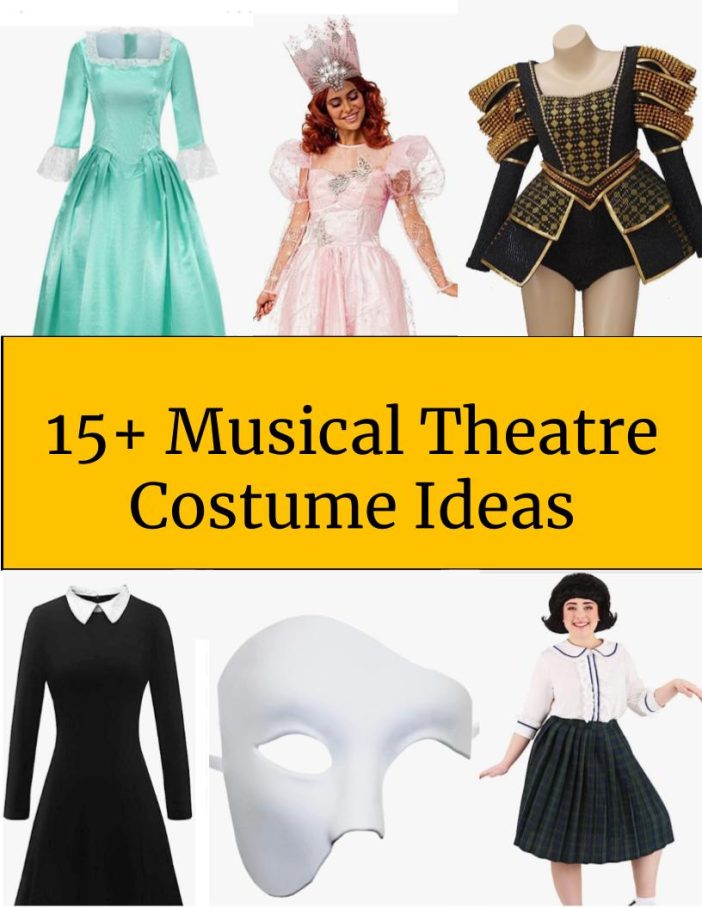The image features a white background with a yellow-bordered center displaying "15+ Musical Theater Costume Ideas" in black font. The top left showcases a turquoise dress with a white collar and cuffs. Next to it in the middle, a woman wears a frilly pink fairy dress adorned with transparent sleeves and gray butterflies, paired with a pink and white crown embellished with pearls. On the top right, a mannequin displays a medieval-looking black dress with gold shoulder accents.

At the bottom left, there's a long black dress with a white collar, reminiscent of something Wednesday Addams might wear. Adjacent to it, a half-white mask evokes the Phantom of the Opera. On the far right, a girl in a black wig models a white blouse and a green plaid long skirt, reminiscent of a school uniform.